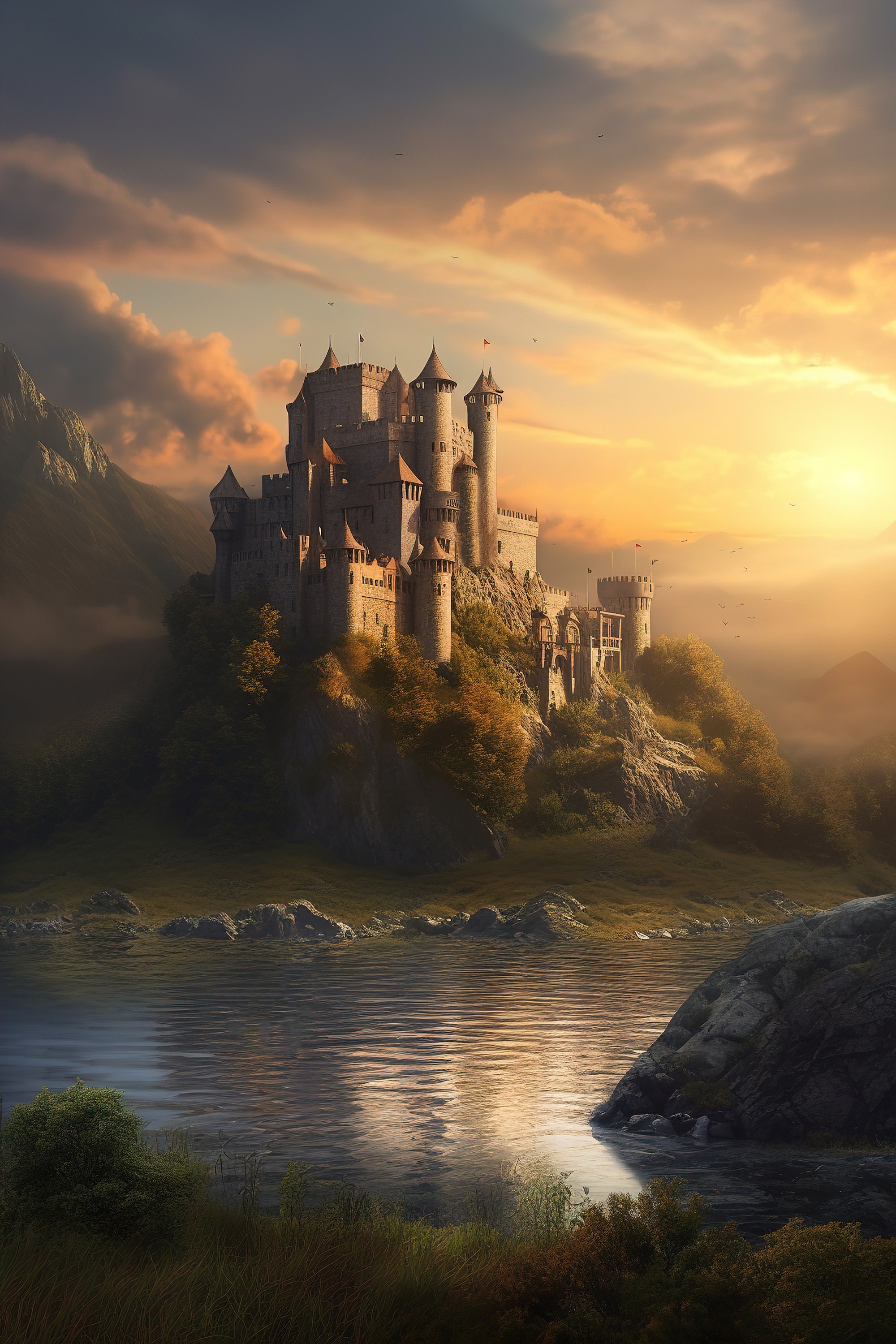The image portrays a hyper-realistic AI-generated painting of a grand 14th-century castle majestically perched on a rocky mountainside. The castle, with its tall towers, crenellations, and mortar holes, stands about 4 to 5 stories high and appears to be built into the mountain itself. It features four or five silo-like turrets, some adorned with colorful pennants fluttering at their peaks. 

The sky above is filled with clouds, interspersed with hints of blue sky and bathed in the warm hues of a setting sun, casting a golden light onto the right side of the scene. The sunlight breaks through the clouds, creating a beautiful gradient of purple, yellow, and pink across the sky.

In the foreground, lush greenery, trees, and climbing vines surround the castle, contributing to the overgrown, ancient ambiance of the scene. At the bottom of the image, a serene moat or stream flows gently by, its crystal-clear water with a few ripples reflecting the tranquil surroundings. A large rock sits prominently in the water near the bottom right of the image, while smaller rocks and more patches of dark green grass pepper the area closer to the castle. Birds fly in the distance, adding a touch of life to this enchanting landscape.